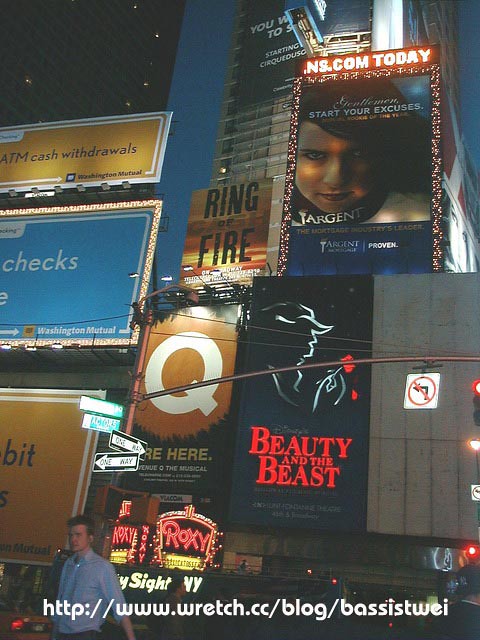This is a nighttime photograph of a bustling city street dominated by towering skyscrapers adorned with a myriad of brightly lit billboards. Prominent amongst the advertisements is the Roxy Theater, glowing in neon, suggesting a possible location in a major city like LA. The scene is lively and crowded with billboards. A central skyscraper features multiple billboards, including "Ring of Fire" and "Beauty and the Beast." Adjacent billboards include one for "NS.com Today" at the top and "Start Your Excuses," featuring a woman's face. Other advertising displays cover diverse topics—one with a menacing little girl for "Tangent," and another for ATM cash withdrawals and checks, showcasing a website at the bottom. The urban setting, saturated with vibrant lights and diverse ads, captures the essence of a place reminiscent of iconic, densely populated areas like Times Square.